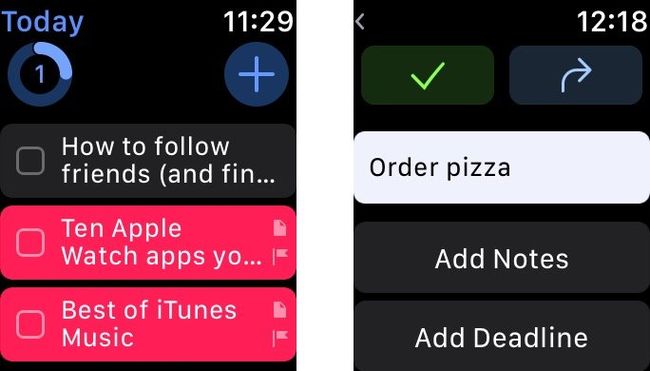This image consists of two different screenshots, likely captured from a smartphone. 

**First Screenshot:**
- **Background & Title:** The top section features a black background with the word "Today" in blue letters.
- **Time Display:** Below "Today," the time is displayed in white letters as "11:29".
- **Highlighted Circle:** There is a partially highlighted circle with the number "1" under the time.
- **Icon:** Beneath this, there is a circle containing a plus sign.
- **Options List:** 
  - The first option reads "how to follow friends," which is displayed against a black background with a small box next to it.
  - The second option is "10 Apple Watch apps" but the text is cut off. The entire area surrounding this option is highlighted in pink.
  - The third option says "Best of iTunes music," similarly surrounded by pink highlighting with small icons on the right side.

**Second Screenshot:**
- **Background & Interface:** The second screenshot also has a black background.
- **Navigation and Time:** At the top, there is a left-facing arrow. On the right side, the time "12:18" is displayed.
- **Green Check Mark:** Below the top bar, there is a green check mark followed by two buttons.
  - **First Button:** The first button doesn’t have a clear label.
  - **Second Button:** The second button features a curved, right-pointing arrow.
- **Order Prompt:** Below the buttons, a white oval bar reads "order pizza".
- **Additional Options:** Under the white oval bar, there are two items: "add notes" and "add deadline".

The images provide a glimpse into a smartphone's interface, showcasing different functionalities, probably related to social interactions and media choices like following friends, exploring apps, and ordering food.